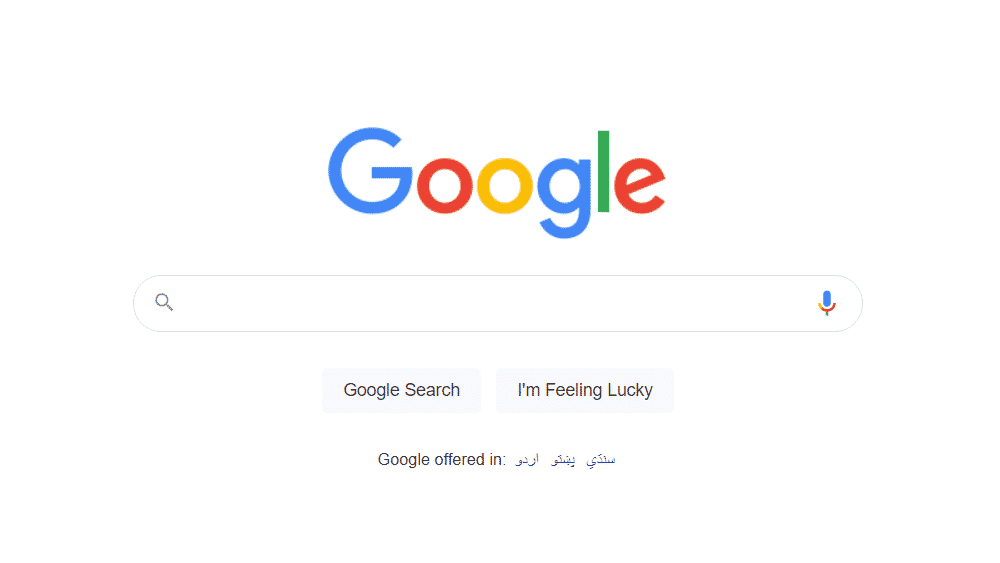The image displays the Google homepage prominently featuring the Google logo at the center top. Below the logo, the search bar is visible, with a microphone icon positioned on the right side of the bar, indicating voice search capability. Underneath the search bar are two buttons: "Google Search" and "I'm Feeling Lucky." Beneath these buttons, there's a notice that reads, "Google offered in," followed by a list of three languages typically associated with regions involved in jihadist activities.